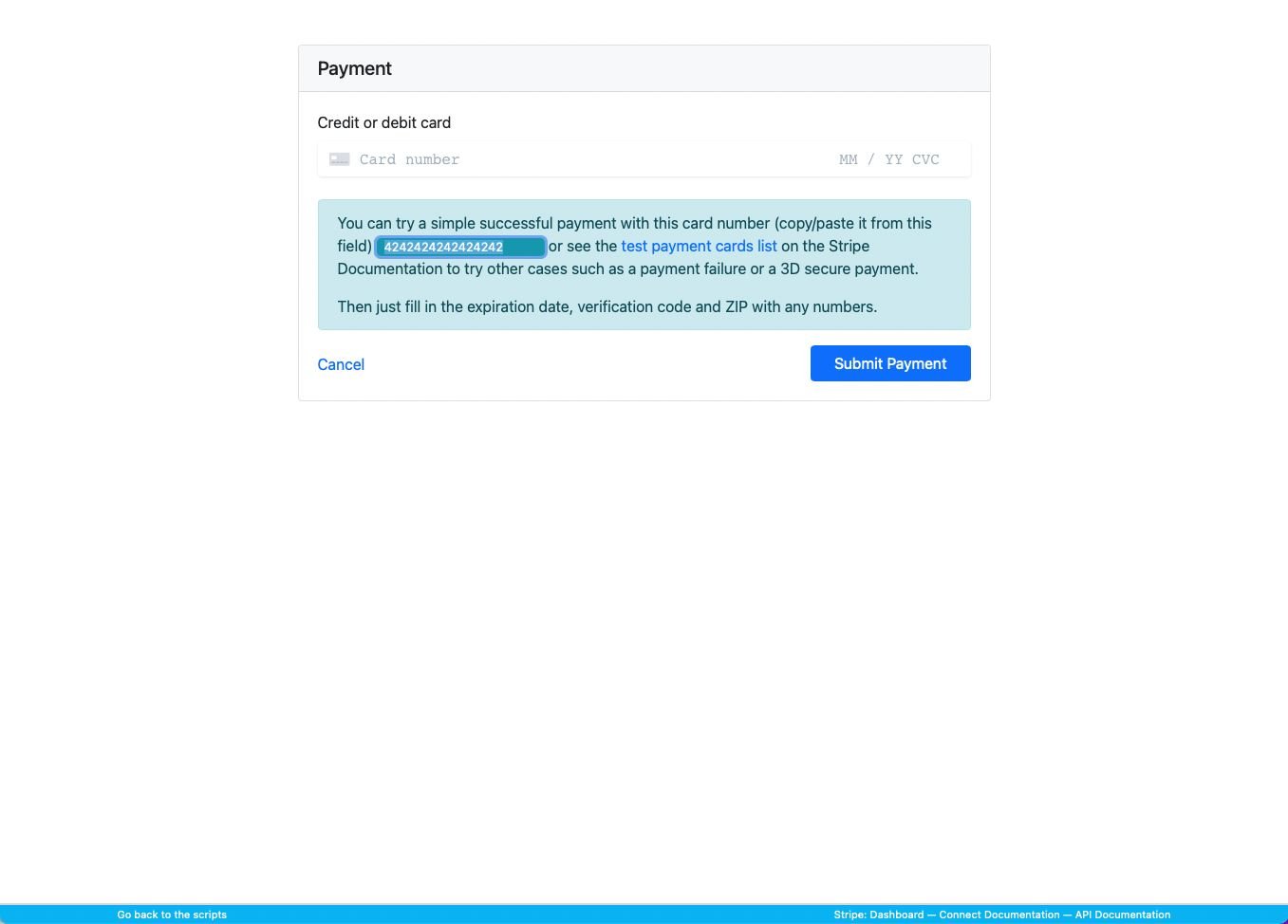The image portrays a payment form interface with various sections aimed at facilitating a credit or debit card transaction. At the top of the form, a grayed-out horizontal rectangle contains the label "Payment" in bold black lettering. Below this, the background remains white with the text "Credit or Debit Card" also in black.

The next section outlines input fields: first is "Card Number" written in gray, paired with a small icon of a credit card to its left. On the far right, the fields "MM/YY CVC" also appear in gray, indicating where users should input their expiration date and security code.

Further down, there is an eye-catching large rectangle box filled with a greenish-blue hue. Inside this box, a bold message of the same color reads: "You can try a simple successful payment with this card number (copy/paste it from this field)."

Immediately following, there's a dark green rectangle containing a sequence of white digits "42 42 42 42 42 42 42 42," suggesting a test card number. Below this, a line in blue text reads: "or see the test payment cards list" which is a hyperlink leading to the Stripe documentation. The additional text guides users to try other scenarios such as payment failure or 3D secure payment by using any numbers for the expiration date, verification code, and ZIP code.

At the bottom of the form, on a white background, to the left is a blue hyperlink labeled "Cancel," while to the far right there is a blue button labeled "Submit Payment" in white lettering.

Finally, at the very bottom of the screen, there is a lengthy blue rectangle. On the left side, it says "Go back to the scripts" in white, and on the right side, it lists various links to Stripe's resources: "Stripe Dashboard," "Connect Documentation," and "API Documentation," all in white lettering.